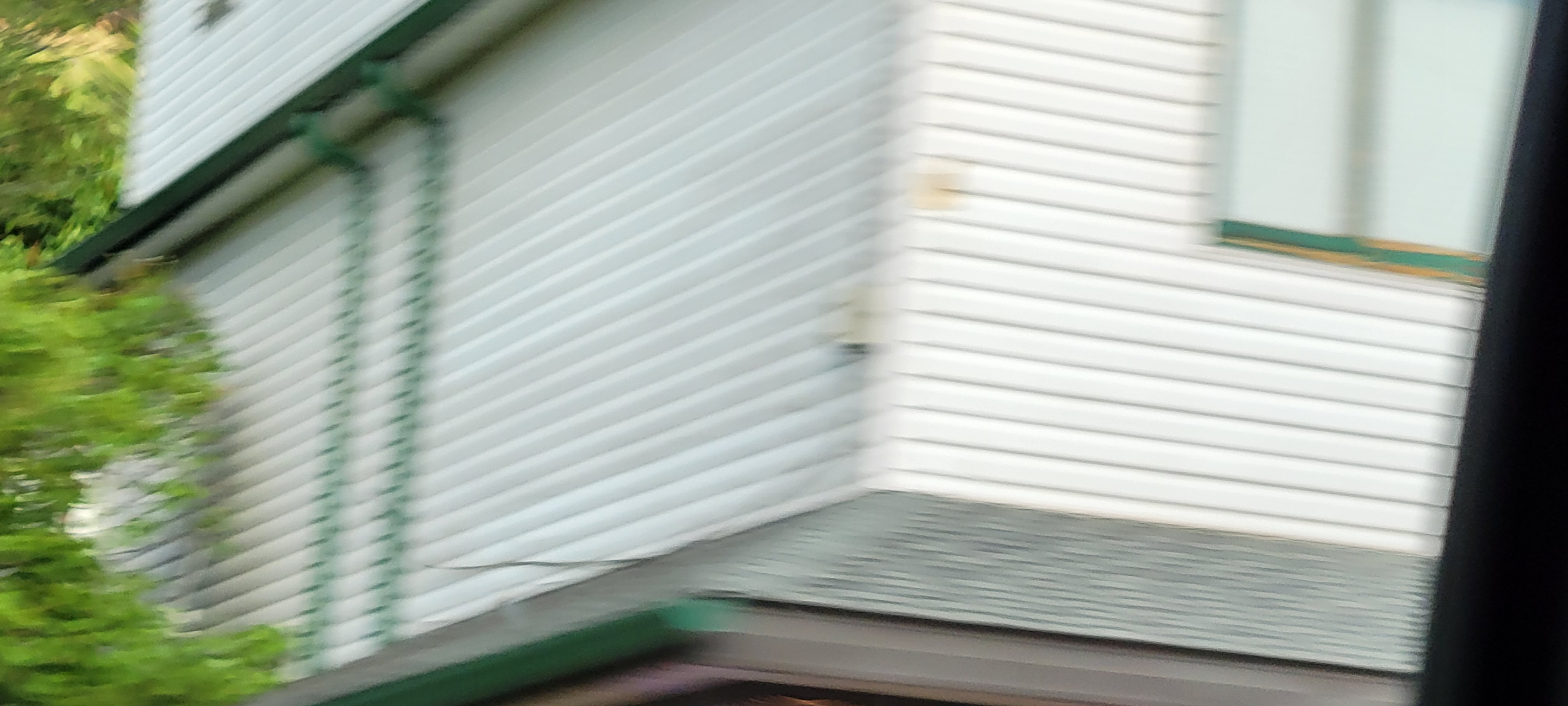This blurry, landscape-oriented image captures the side of a modern, three-story house with white horizontal siding and a greyish roof. Accents of green piping or eaves trough run down the left side, with additional green eaves troughs around both the garage roof and the top roof above the second story. At the top right of the image, there's a window featuring green frames on the inner and outer edges, with a mix of green and orange at the base and brown trim. The window appears to have shades drawn, obscuring the interior. The left side of the image is dominated by greenery, with tree branches extending towards the house. There are no people or text in the image, and the overall aesthetic suggests a clean and modern design, despite the photo's blurriness.